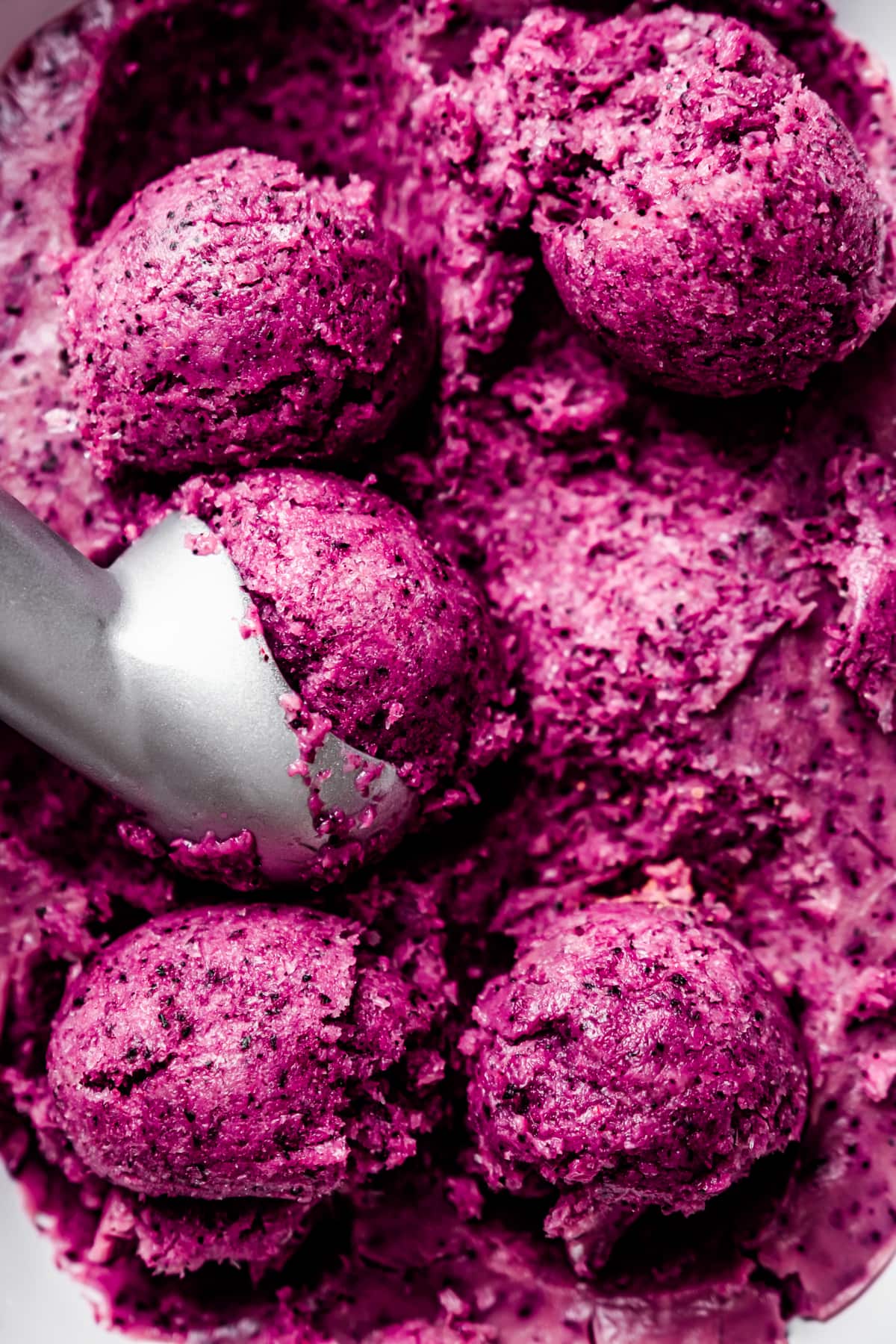A silver scooper, positioned from the left center edge of the image, is seen in the act of forming a ball of dark purple ice cream with reflective white sheen and black specks. This scoop is extracting the ice cream from a dish. There are five balls of this purple ice cream visible in total, arranged neatly with two above the scoop, two below, and one being scooped. The ice cream's dark purple color is prominent, with potential chocolate sprinkles adding texture. The image showcases the detailed process of preparing and arranging the ice cream for serving.